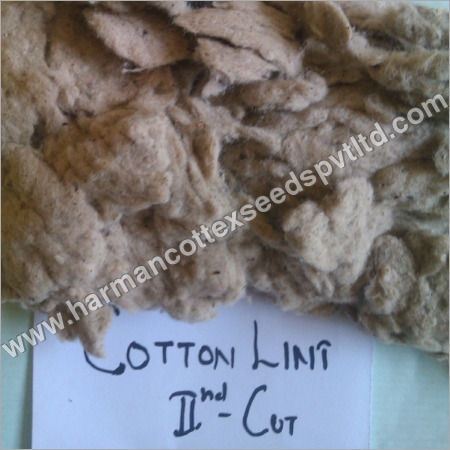In this image, a large, lumpy pile of grayish cotton lint occupies the top two-thirds of the frame. The lint forms numerous clumps, giving it a fluffy texture. At the bottom of the image, there is a white piece of paper with handwritten black letters that clearly read "Cotton Lint." Below this label, the paper features the inscription "Second," using Roman numerals (II), followed by "C-O-T." This piece of paper rests on a dull teal tablecloth. Additionally, a transparent watermark with the text "www.harmancottexseeds.com" is angled diagonally from the lower left corner to the upper right corner of the image.